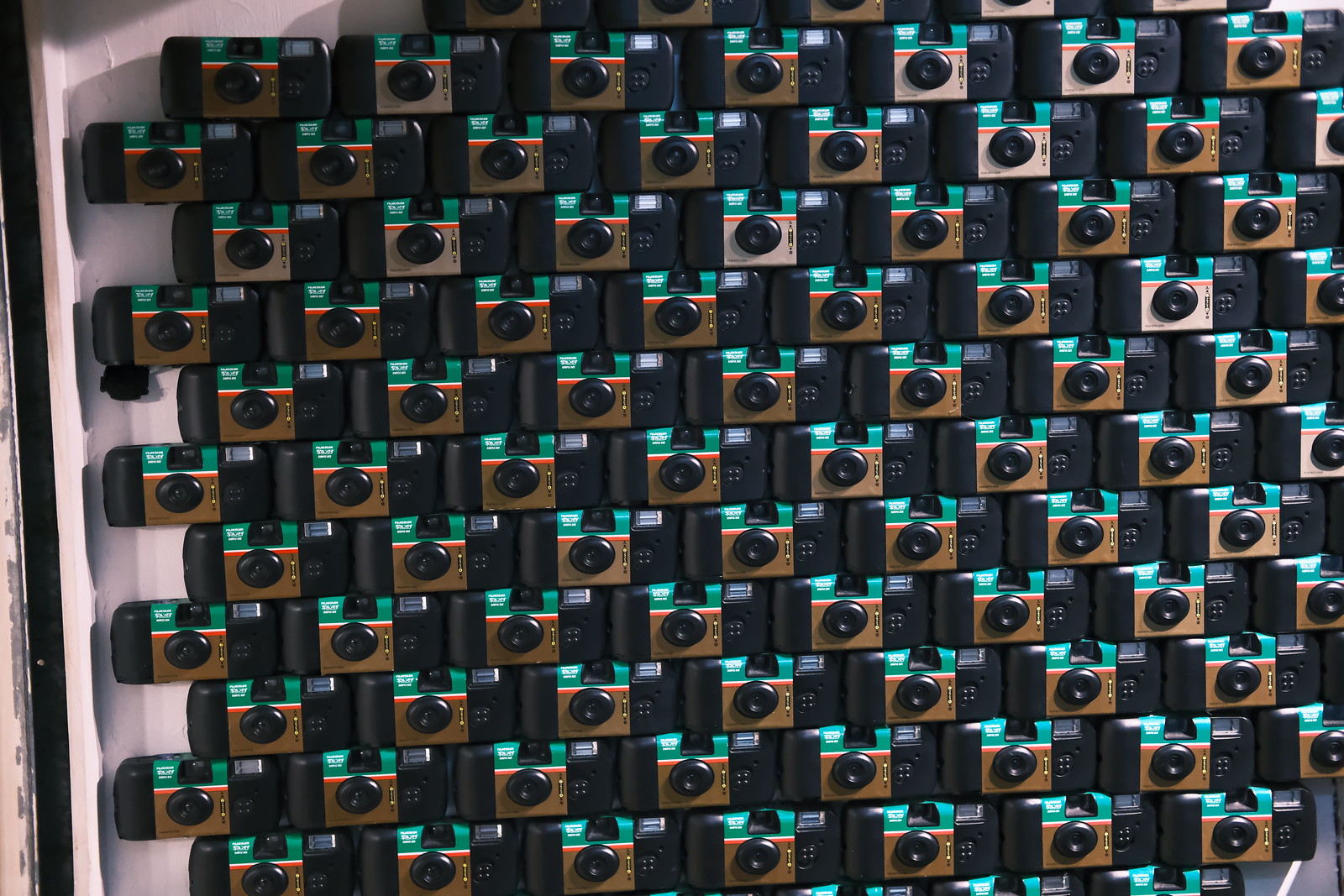This photograph captures an artistic installation featuring a wall meticulously covered with approximately 80 to 100 identical 35mm cameras. Each camera is uniquely characterized by a black outer casing, a brown square in the middle with a lens set at the top, and a green upper section boasting a central viewfinder. There's a small, indistinct white detail on the left side of the green section. The cameras are expertly arranged in a brick-like or checkerboard pattern against a predominantly white wall with some subtle black elements visible. The varying light reflections and a touch of sunlight in the lower right corner emphasize the physical presence of the cameras, confirming that this is not a digital representation. Additionally, a black bar on the far left suggests the possibility of a window, though it’s partially obscured. There's also a mysterious black element protruding from behind one of the cameras in the upper left, which might be an exposed part, such as a battery compartment.